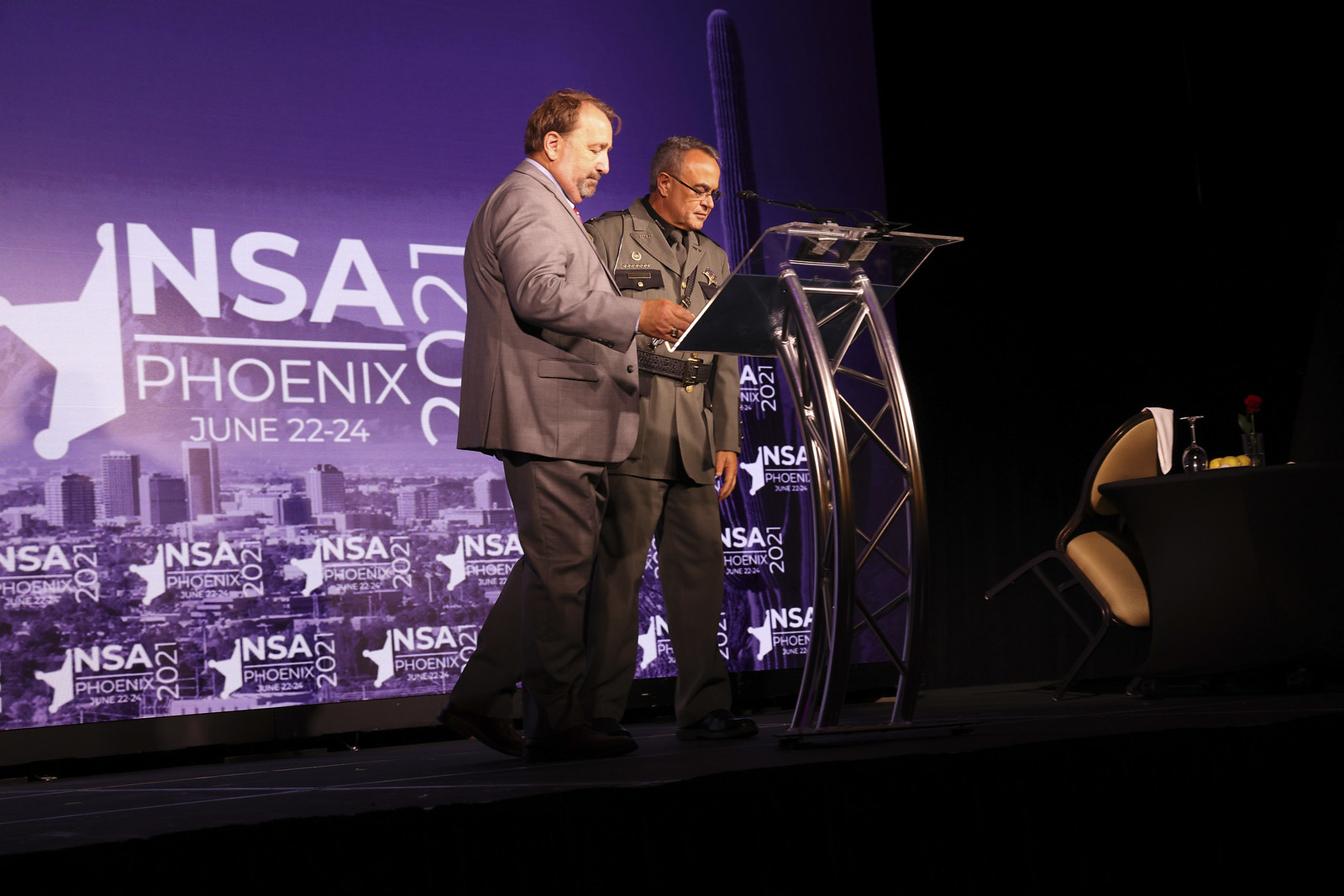The horizontally-oriented photograph depicts two men, seemingly in their 40s, standing on a stage behind a sleek, curved metallic lectern with an angled surface. Both are dressed in brown suit jackets and darker brown pants. The man on the right is wearing glasses. They are engrossed in reading something from the lectern. The background features a prominent banner adorned with purple and white colors. The banner showcases white text that reads "NSA Phoenix, June 22nd-24, 2021," with "2021" displayed vertically on the right. The left side of the banner includes a half star emblem, and beneath the text is a repeated pattern of the "NSA Phoenix 2021" logo accompanied by an outline of the city of Phoenix. The bottom part of the photo is dark, with an indistinct object, possibly chairs, visible to the right, suggesting an awards ceremony setting. The scene is adorned with dim lighting that highlights the men and the lectern, while casting softer light around the stage and background.